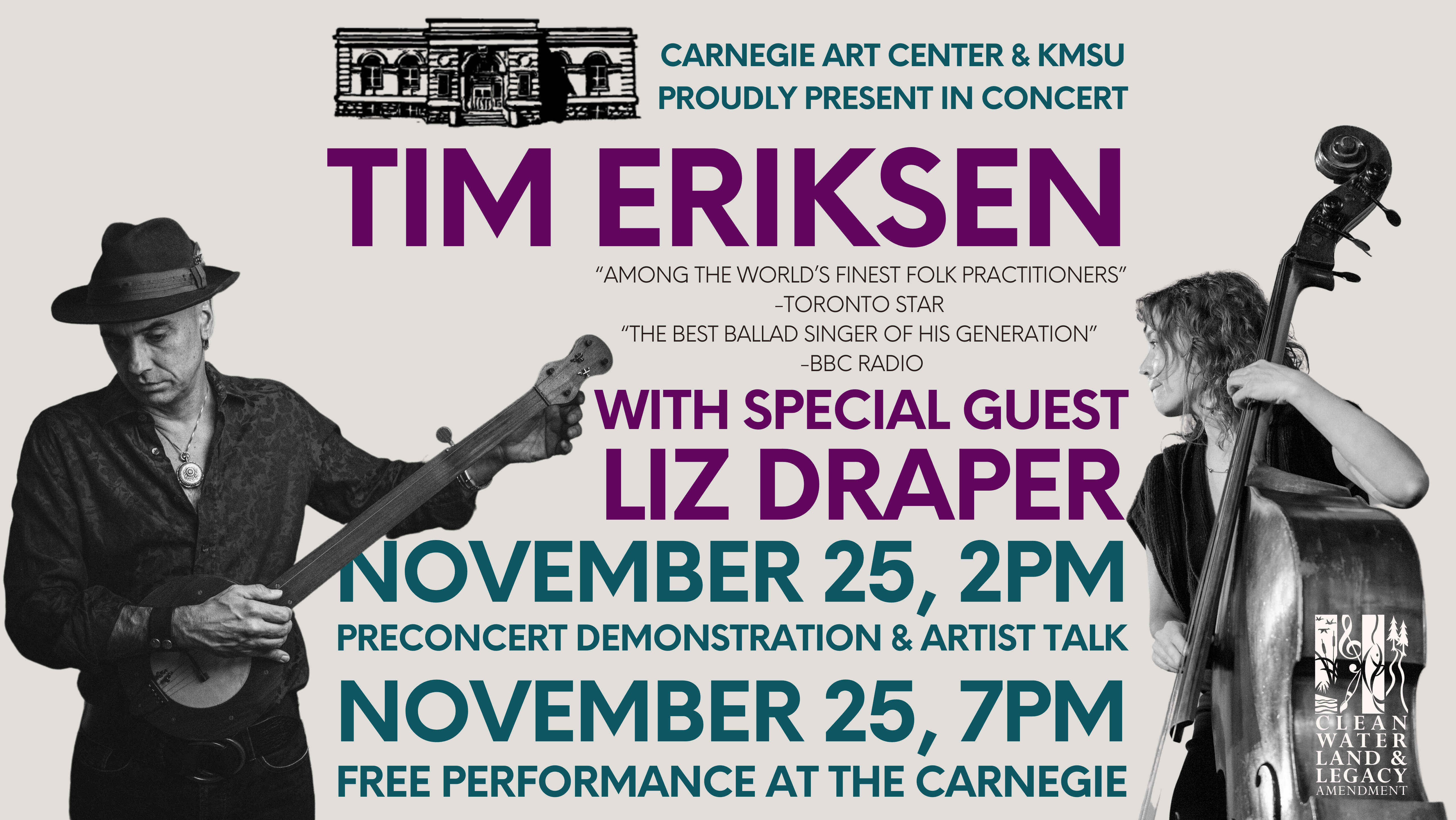This poster, advertising a musical event at the Carnegie Arts Center, proudly presented by KMSU, features Tim Erickson and special guest Liz Draper. In black and white, the poster showcases a photograph of Tim Erickson, renowned by BBC Radio as the "best ballad singer of his generation," playing a small banjo-like instrument and wearing a brimmed hat. Beside him is Liz Draper, celebrated in folk circles, standing with a large bass, often referred to as a bass fiddle. The event details are highlighted in vibrant purple and green text, indicating two performances on November 25th at 2 PM and 7 PM, both incorporating a free concert, demonstration, and artist talk. The poster includes a black-and-white drawing of the Carnegie Arts Center building, emphasizing its significance in hosting this distinguished folk music event.